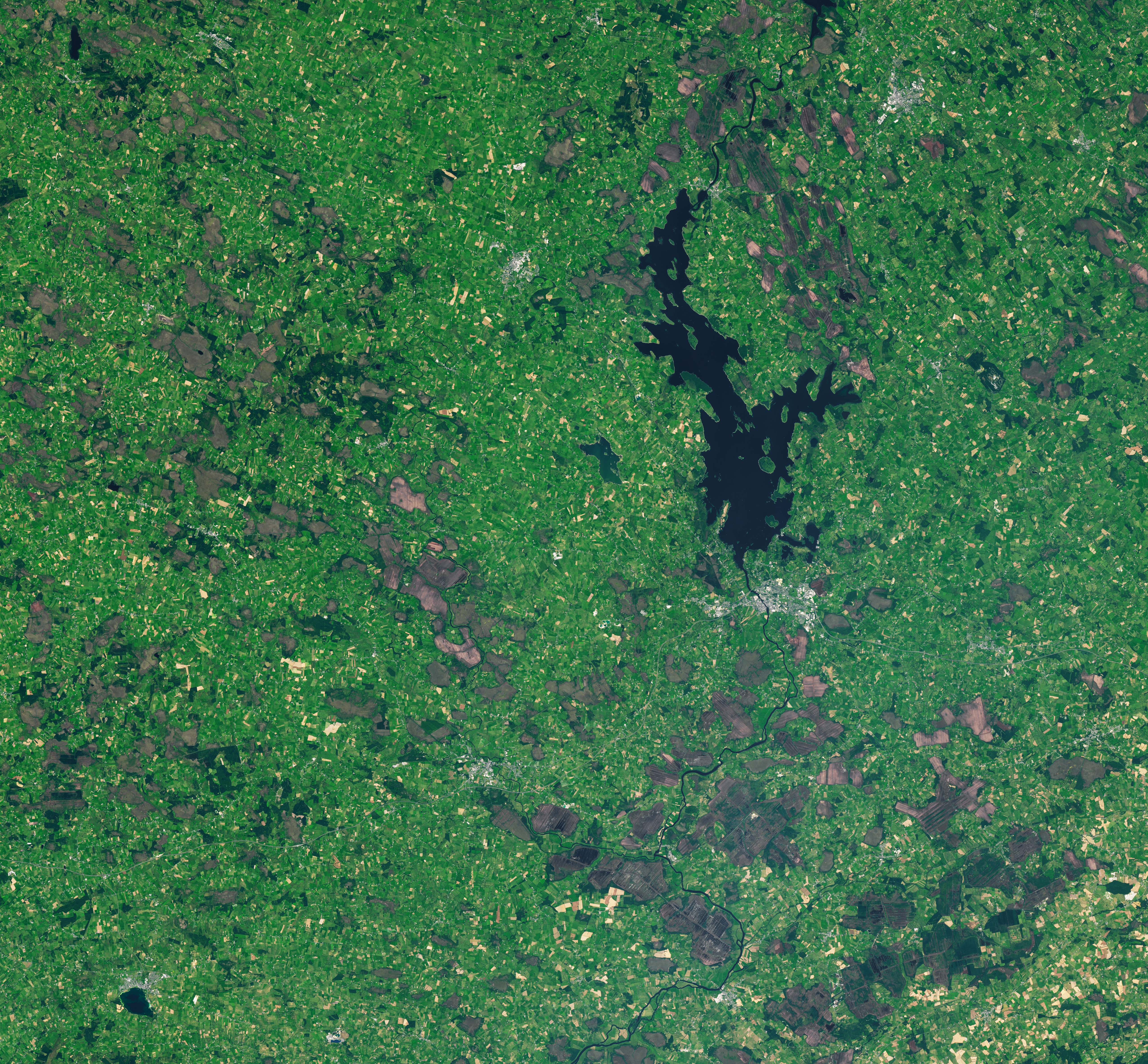The image is a square, predominantly filled with various shades of green, evoking a flat, grassy expanse. Scattered throughout are specks and highlights in black, gray, brown, and tan, giving it a somewhat peppered appearance. At the center-right, there is a prominent black blotch with branching extensions, resembling either an aerial view of a lake or some abstract form. These shapes and colors blend organically, potentially suggesting a natural landscape, but there's ambiguity about the exact nature of the image—is it an aerial photograph, a microscopic view, or a piece of abstract art? The lack of any text, borders, or other enclosures, along with the mix of tones and shapes, adds to the visual intrigue and leaves its true purpose and origin open to interpretation.